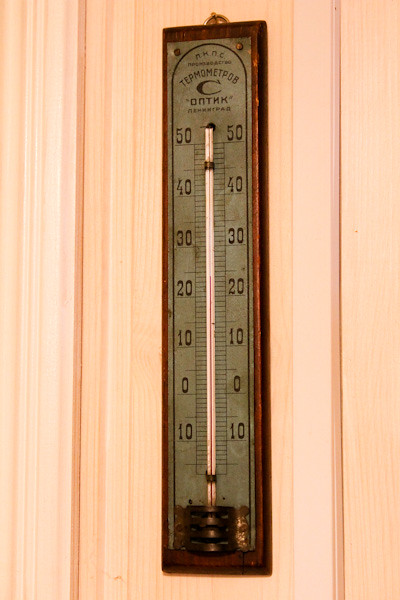A vintage mercury thermometer with Cyrillic inscriptions is prominently displayed against a backdrop of fresh, bright pine wood. The thermometer, encased in a discolored metal housing, features a glass tube filled with mercury and is marked by the numbers 50, 40, 30, 20, 10, 0, and -10 degrees on both sides, each separated by precise striations. It hangs from a well-worn brass hook attached to a corroded metal base with four decorative bars wrapping around it. The pine wall, constructed from various strips of batten, trim, and molding, is illuminated by a direct light source from the left, casting a brighter light on the left side of the image and gradually dimming toward the right. The photograph captures the texture and clarity of the wooden background in high resolution, contrasting with the slightly blurred and less detailed rendering of the thermometer itself.